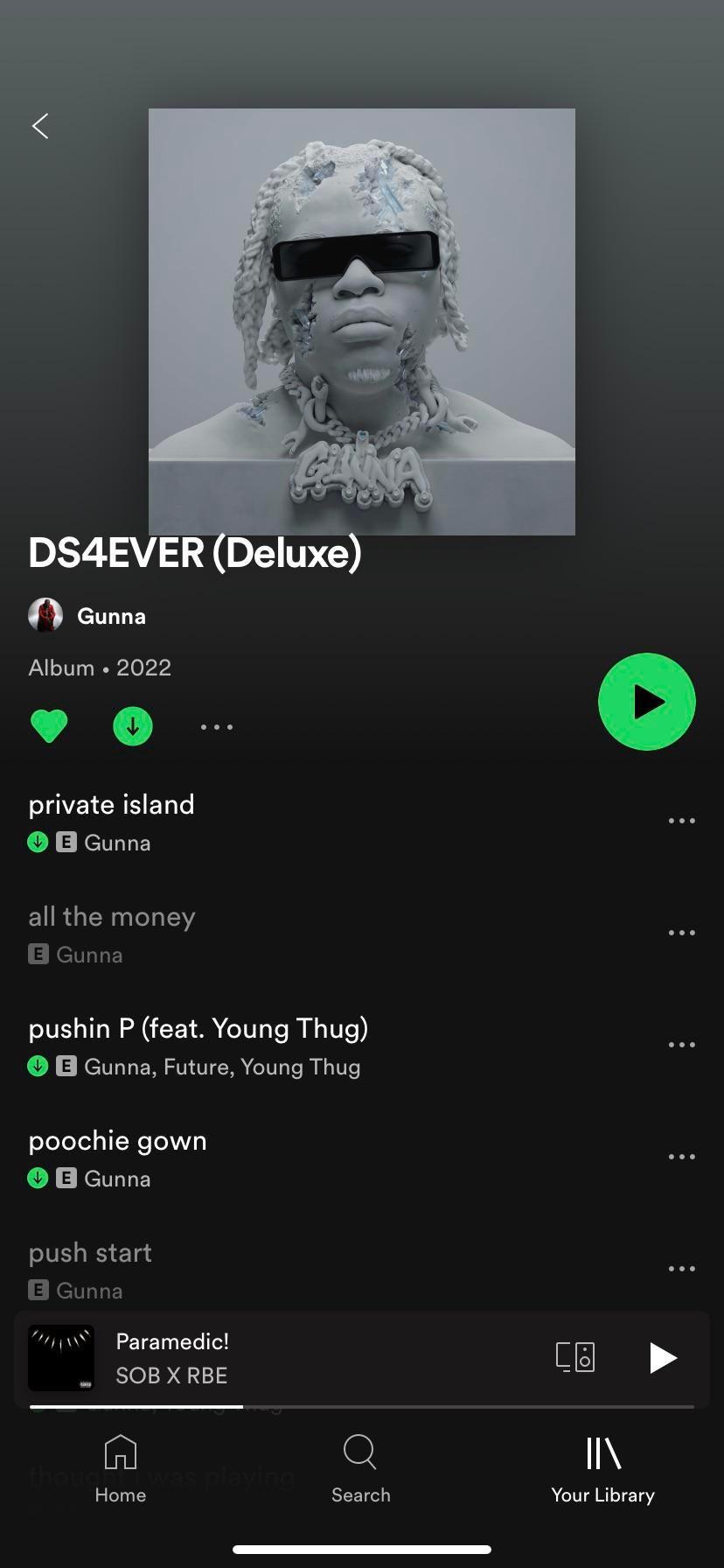The image is a vertical mobile screenshot featuring a music streaming app with a sleek, gradient background transitioning from dark gray at the top to jet black at the bottom. At the top center is an album cover that is predominantly black and white with touches of blue. The cover art depicts a sculpture of a head adorned with long, ringlet hair and wearing a distinctive black-panel-like pair of sunglasses. A necklace on the sculpture reads "CHINA." Below this, the text "DS4EVER (Deluxe)" is displayed on the left. 

The artist's name, "GUNNA," is prominently shown along with a small profile picture and the album’s release year, "Album 2022." Accompanying this information are a heart icon, a download icon, and a play button, all highlighted in green. 

The tracklist is displayed below, featuring songs in order: "Private Island," "All the Money," "Pushin' P" (featuring Young Thug), "Poochy Gown," and "Push Start." 

At the bottom banner, the currently playing song is "Paramedic," accompanied by a right-pointing play button and several other control icons. Further down is the app's navigation bar, which includes a home button, a search button, and a "Your Library" button. A centered white horizontal line at the footer bar completes the layout.